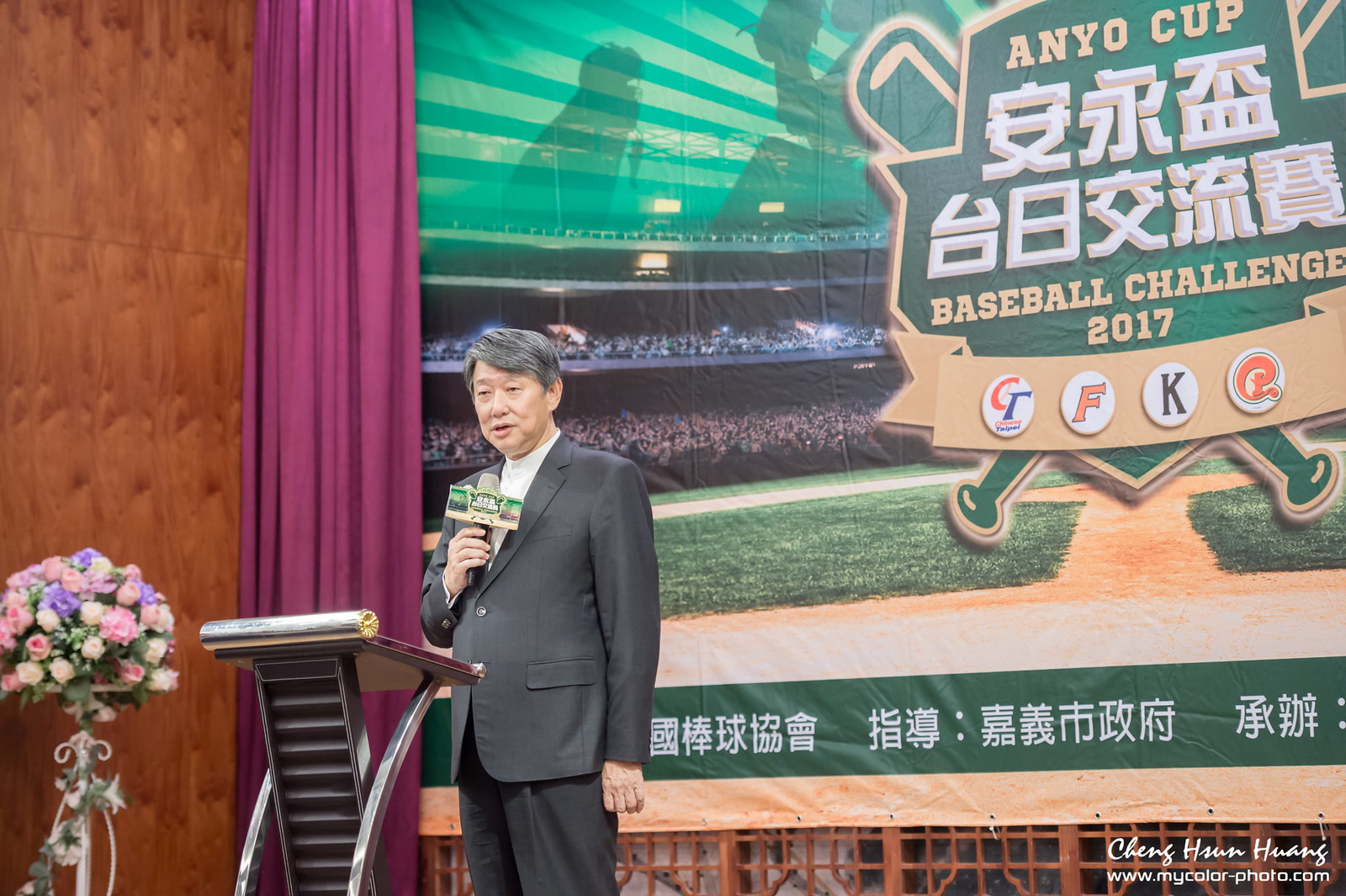This indoor photograph, taken in landscape mode, captures a stage setup for the Anyo Cup Baseball Challenge 2017. Central to the image is an older Asian man with graying black hair, dressed in a gray suit and white button-up shirt, standing at a podium while speaking into a microphone. The microphone features event branding at its top. The man is positioned slightly to the left of the image center, illuminated against a backdrop of various colors including purple, pink, yellow, and green.

Behind the speaker, there is a large tarpaulin banner with an image of a baseball field from the perspective of home plate. Prominently displayed in the center of the banner is a green shield with a gold outline, flanked by crossed baseball bats. Inside the shield, "Anyo Cup" is written in gold print, followed by Asian script and the English text "Baseball Challenge 2017." Below these inscriptions, the graphic features four sports team logos spread across a ribbon. 

To the left of the banner, a row of bunched-up pink curtains descends from the top of the image, juxtaposed against a brown wooden wall on the left-hand side. In the lower left corner, there is a meticulously arranged bouquet of pink, purple, and white flowers on a white stand. The lower right corner bears a cursive signature, "Chang Sun Hwang," along with the URL www.mycolor-photo.com.